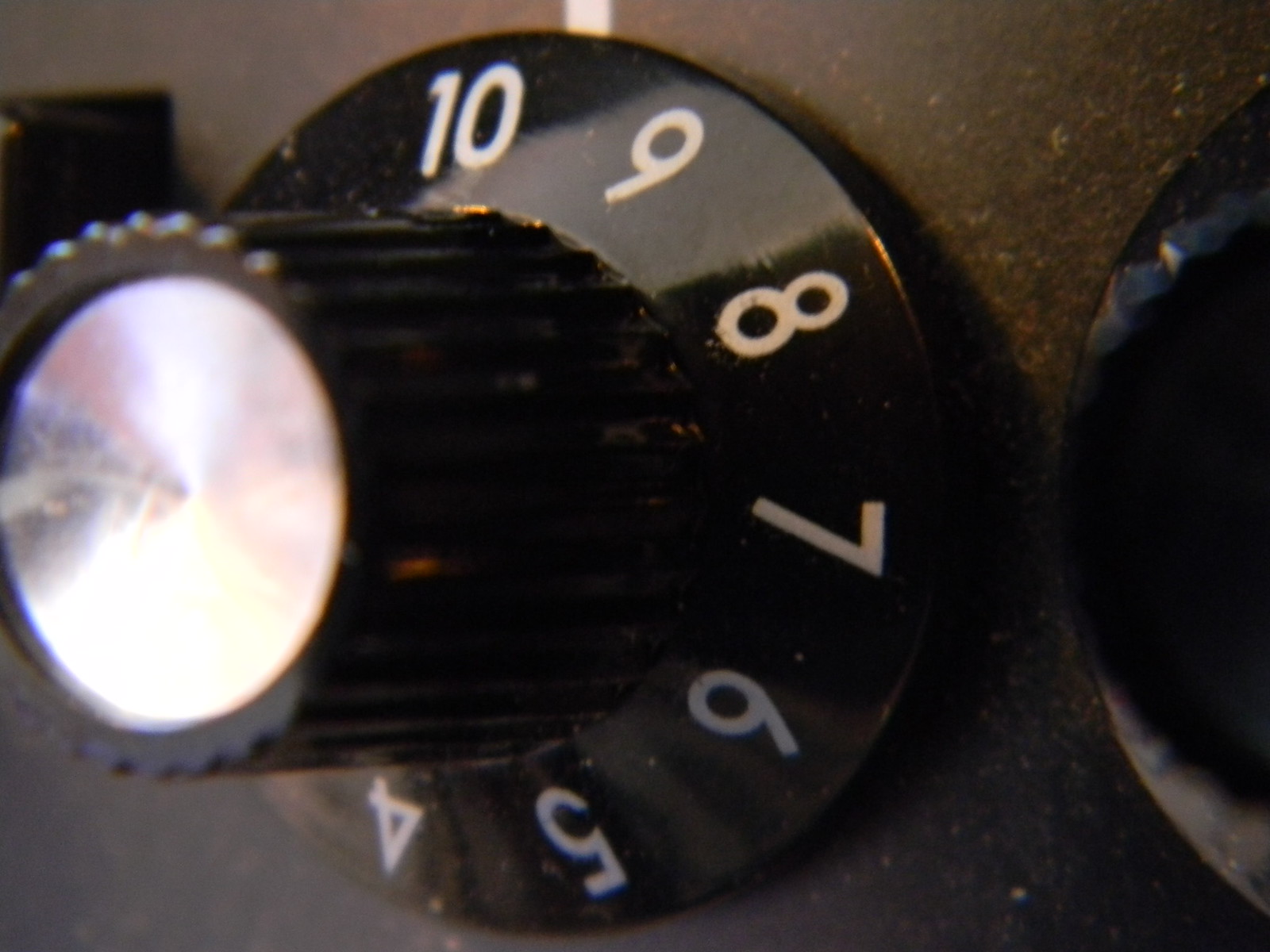The image showcases a close-up view of a black oven knob, prominently positioned at the top center of the picture. The knob is circular and features distinct white numbers arranged in a counterclockwise direction from 10 down to 4, with the numbers 3 to 1 obscured by the knob itself. The design includes a cylindrical shape with ridged edges for grip, and its flat center has a silver metallic surface. The knob is mounted on a black dashboard surface, which appears slightly grimy with traces of white dust. Adjacent to this knob, there is a hint of another knob on the right and an indistinct square object to the left on the dark, possibly grayish-black, background. The numbered markings are clear and not peeling, providing a sharp contrast against the knob's black body.